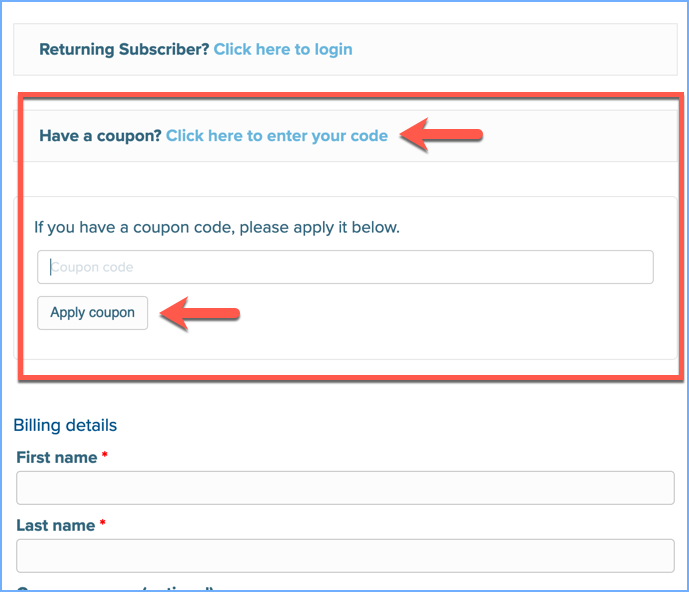In this image, the design starts with a vibrant blue outline against a clean white background. Below this, there is a light grey box containing text in a gradient from dark to light blue font, posing the question "Returning subscriber?" and prompting with "Click here to log in" in light blue font.

Adjacent to this, an orange-outlined, light brown box provides an option with the heading "Have a coupon?" combined with a clickable link that encourages users to "Click here to enter your codes." This section is accentuated by a red arrow pointing directly at it for emphasis.

Separating this from the next section is a visible dividing line. The subsequent box displays text instructing, "If you have a coupon code, please apply it below," in light grey font. Underneath is a text field labeled "Coupon Code," which consists of a white input box for typing in the coupon. Flanking this input is a button labeled "Apply Coupon" in blue font set against a white background. This area is highlighted by an orange arrow for easy identification.

Outside the orange-outlined box, there is blue lettering that reads "Billing Details." Directly below this header, in darker font, labels for "First Name" and "Last Name" appear, each marked with a mandatory red star. Adjacent to these labels are light grey boxes designated for filling in personal details. The form concludes with another section marked by a red outline at the bottom of the page.